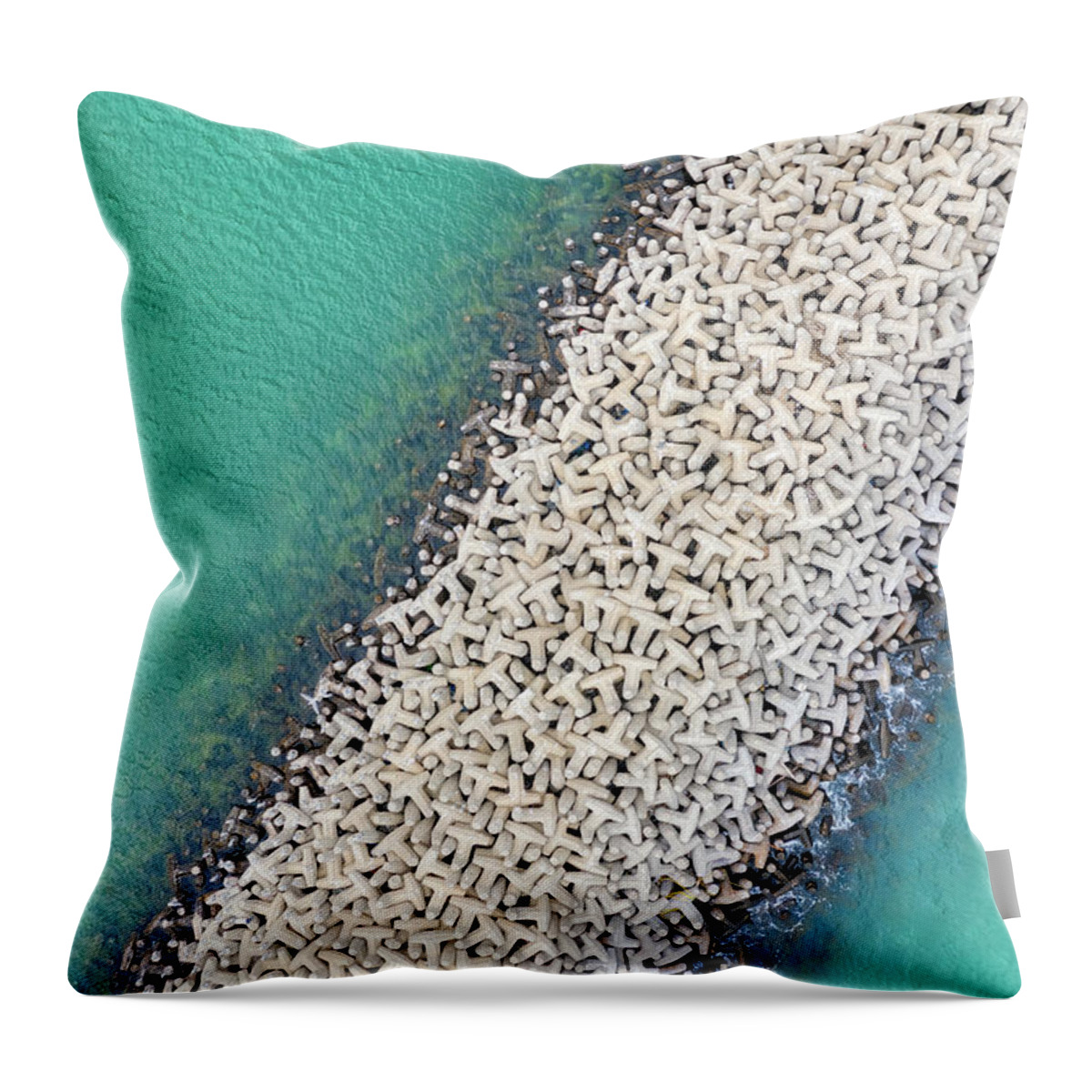This photograph features a close-up of a throw pillow set against a white background. The pillow displays an abstract, vivid turquoise design that gives the impression of a scene involving water and shorelines. At its core, the pillow is adorned with a series of T-shaped objects resembling bones or tile spacers, which appear to form a cascading pattern from the bottom left to the top right corner. The color palette transitions from deep aqua and teal shades at the corners, becoming lighter and more mixed towards the center. These T-shaped details vary in color, appearing tan or sand-like in the dryer areas and darker brown in the regions that might represent wetter conditions. Some of these shapes seem to be falling into the sea, creating splashes, especially noticeable towards the bottom right corner of the pillow. The intricate design captures an essence of movement and depth, with the water appearing translucent in parts and exhibiting gentle waves. The pillow also includes a tag, subtly visible on the back.